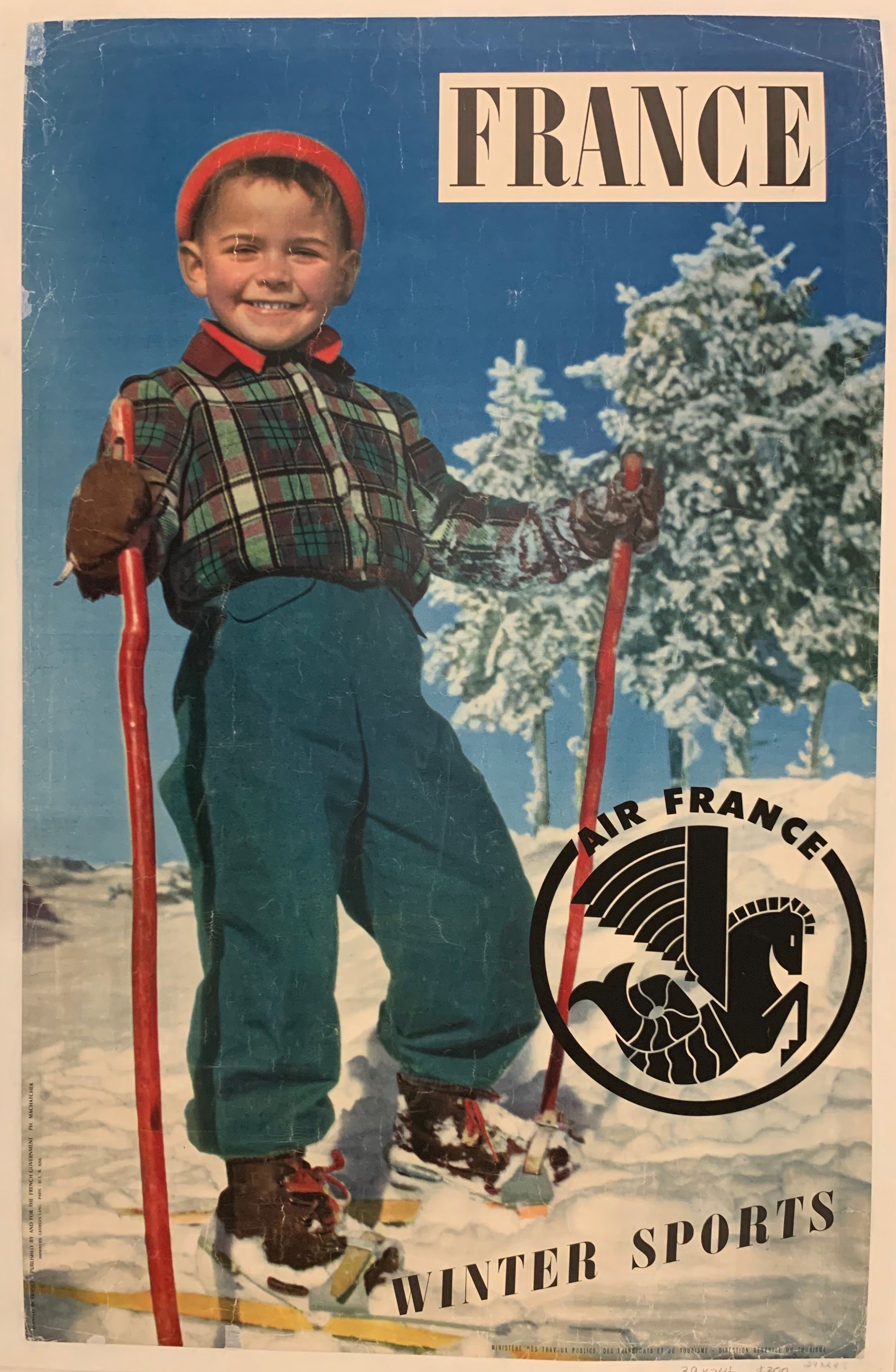The image appears to be an old magazine page or travel poster, likely from 20 to 30 years ago, featuring an advertisement for Air France and winter sports. At the top of the page is the word "France" in bold black letters against a beige background. Below, on the right side, is a black circle with the Air France logo, resembling a pegasus, inside it. Just beneath the logo, the text reads "Winter Sports."

In the snowy scene, a cheerful young boy, around 6 to 8 years old, stands with skis on his feet. He wears a red knit cap, a flannel shirt with an evergreen color interspersed with red and white checks, brown gloves, and green pants. The boy’s brown ankle boots are partially covered by his yellow skis, and he grips red ski poles in his hands. The background showcases a snow-covered hill dotted with evergreen trees dusted in snow, under a clear blue sky. The overall image exudes a nostalgic charm and promotes the joy of winter sports in France, possibly hinting at the services offered by Air France for such travel adventures.